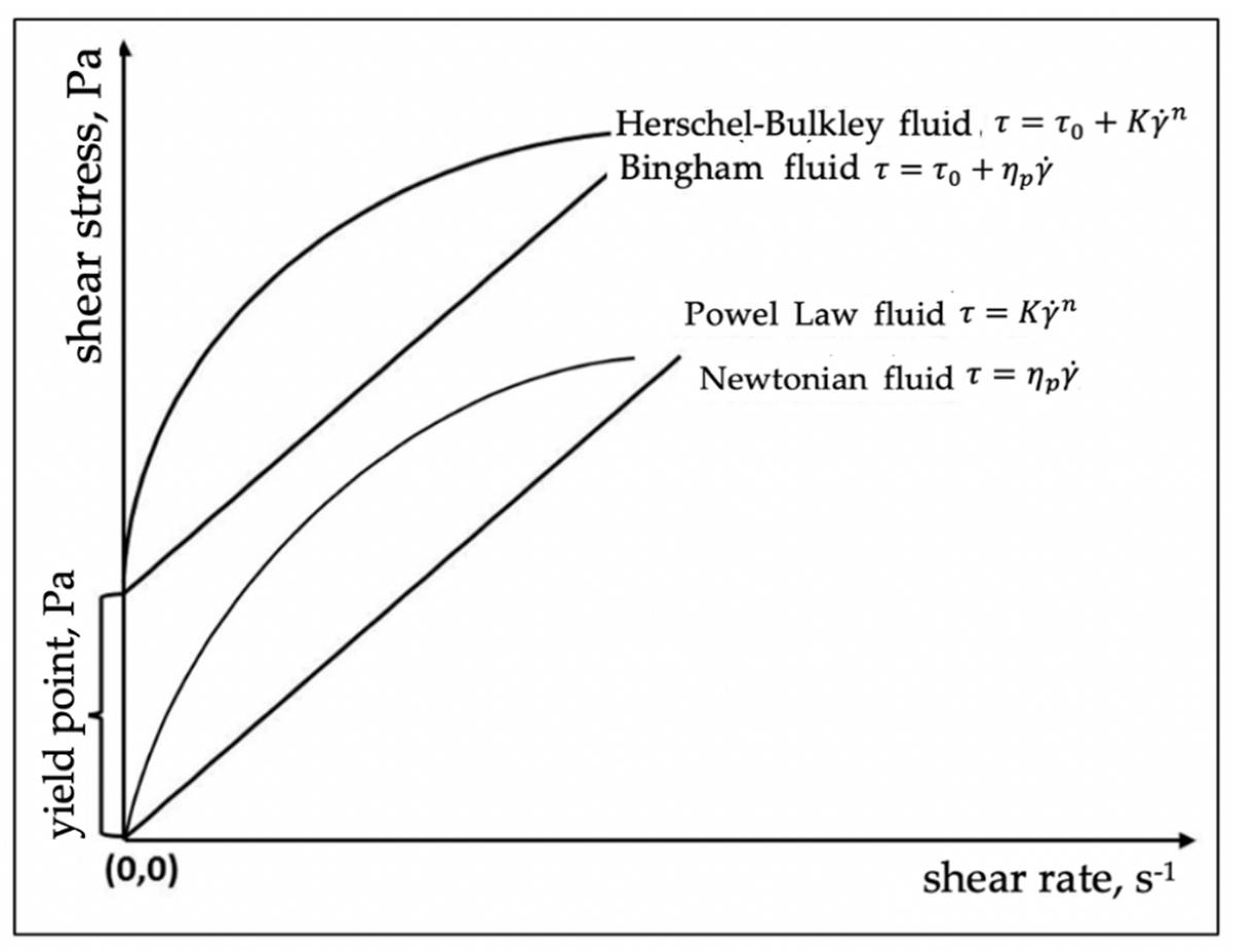This black-and-white image depicts a detailed mathematical graph focused on different fluid behaviors. The graph features an x-axis labeled as "Shear Rate (s⁻¹)" and a y-axis labeled as "Shear Stress (PA)," with the origin at (0, 0). Text on the left side also mentions "Yield Point (PA)." The graph includes four distinct lines representing various fluid models. 

1. The **Newtonian fluid** is shown by a straight diagonal line, described by the equation \( \tau = \eta \dot{\gamma} \) and passing through points like (1, 1), (2, 2), (3, 3), etc.
2. The **Power-Law fluid** curves upward and follows the equation \( \tau = K \dot{\gamma}^n \).
3. The **Bingham fluid** is depicted by a straight line that begins at a certain yield stress value and maintains a linear relationship, described by \( \tau = \tau_0 + \eta_P \dot{\gamma} \).
4. The **Herschel-Bulkley fluid** is represented by a curved line above the Bingham fluid, following the equation \( \tau = \tau_0 + K \dot{\gamma}^n \).

Each fluid type is clearly labeled with its corresponding mathematical formulas, illustrating the different stress-strain relationships inherent to each fluid model. The image efficiently conveys these complex relationships through its clean layout and clear labels.